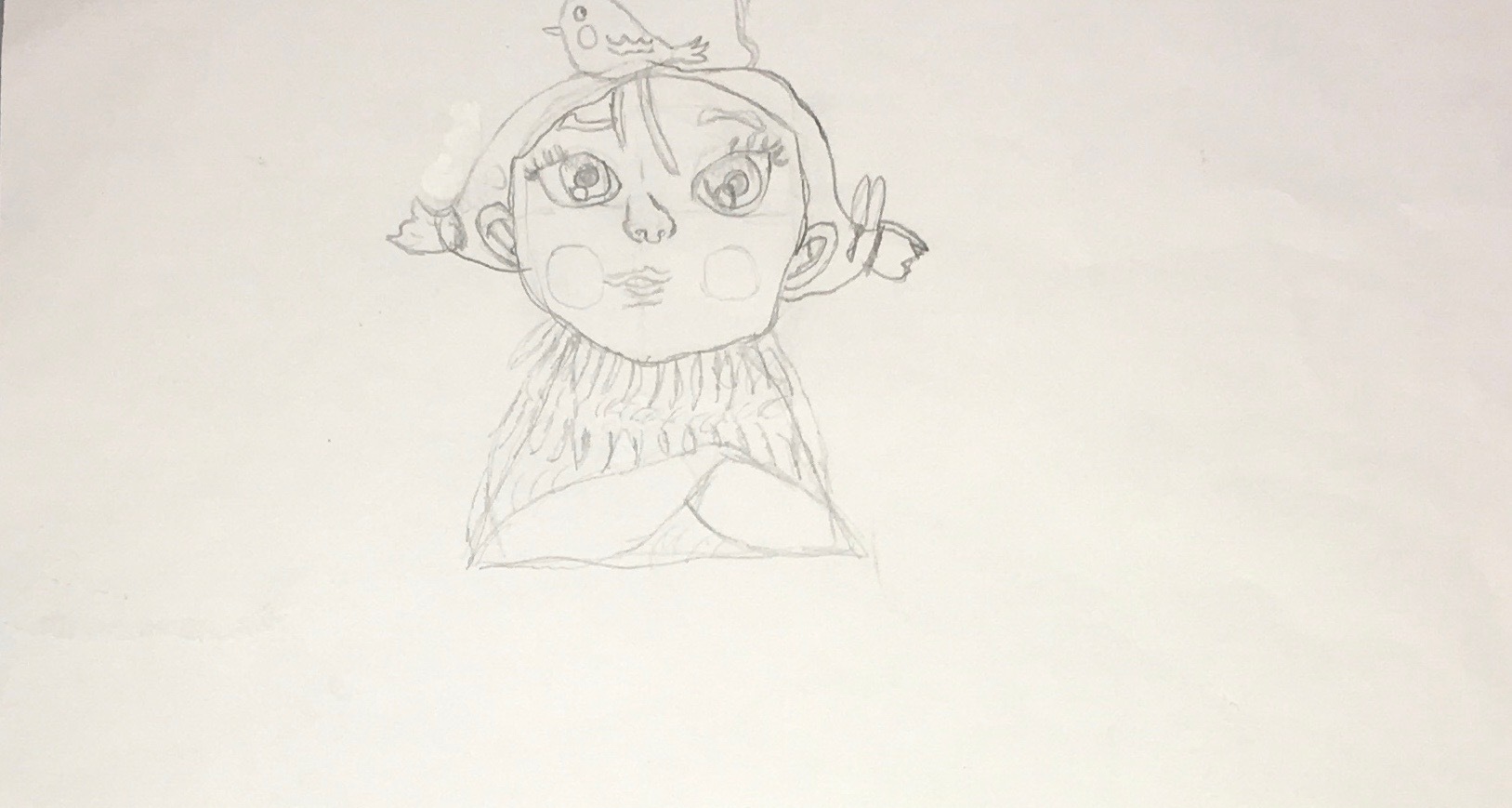This pencil sketch, meticulously crafted on paper, features a line drawing void of color or shading, potentially rendered in either pencil or a very light blue pen. Centered on the page, the artwork portrays a young girl characterized by her large, expressive eyes, pronounced eyebrows, and a discernible nose. Delicate circles embellish her cheeks, suggesting a blush. Captured from the waist up, she sits with her arms crossed, exuding a contemplative aura. Her hair, parted neatly in the middle, cascades down near her ears, where it is tied into pigtails with charming bows. Perched atop her head is an unusual little bird, depicted in profile with its wings folded, exuding a sense of serene contentment. Both the girl and the bird maintain a composed, unsmiling demeanor, quietly sharing a moment of mutual existence.